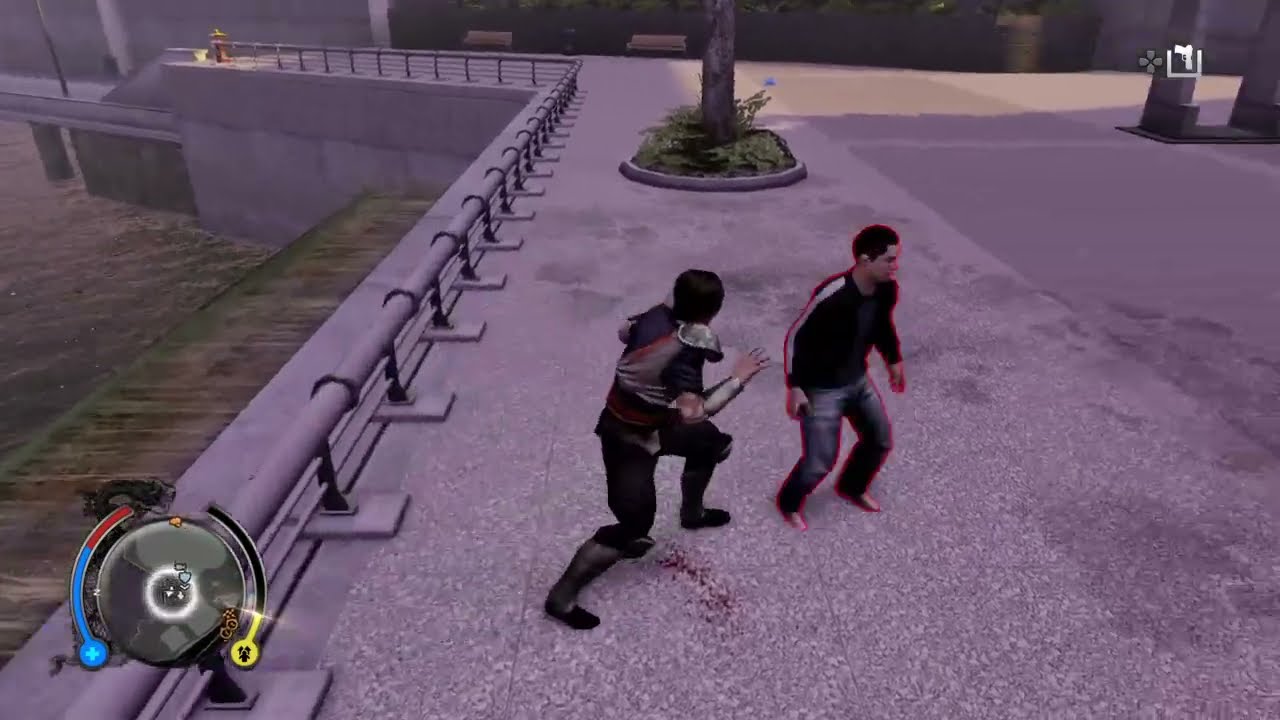This horizontal, rectangular image appears to be a still shot from a video game. The setting suggests a city environment, possibly near a bridge or park, with visible park benches, trees, grass, and a river. In the upper right-hand corner, there is a road adjacent to a sidewalk that transitions into a wooden platform. A metal border wall on the left side suggests they might be on the top of a pier, with water visible below, potentially flowing over a dam. 

In the center of the image, two characters confront each other. The character on the left, donning black pants, boots, and silver armor on their arm and neck, is lunging towards the character on the right, who is dressed in jeans and a black, long-sleeved shirt with stripes. This male character appears to be preparing to evade with his body slightly turned to the right, outlined mysteriously with a red glow. Below this character is a blood splatter, indicated by red dots. 

In the lower left-hand corner, there is a circular interface icon displaying two curved bars; one bar transitions from red to blue with a plus sign, possibly indicating health, while the other transitions from black to yellow. The background is largely devoid of other characters, highlighting the tension between the two central figures.